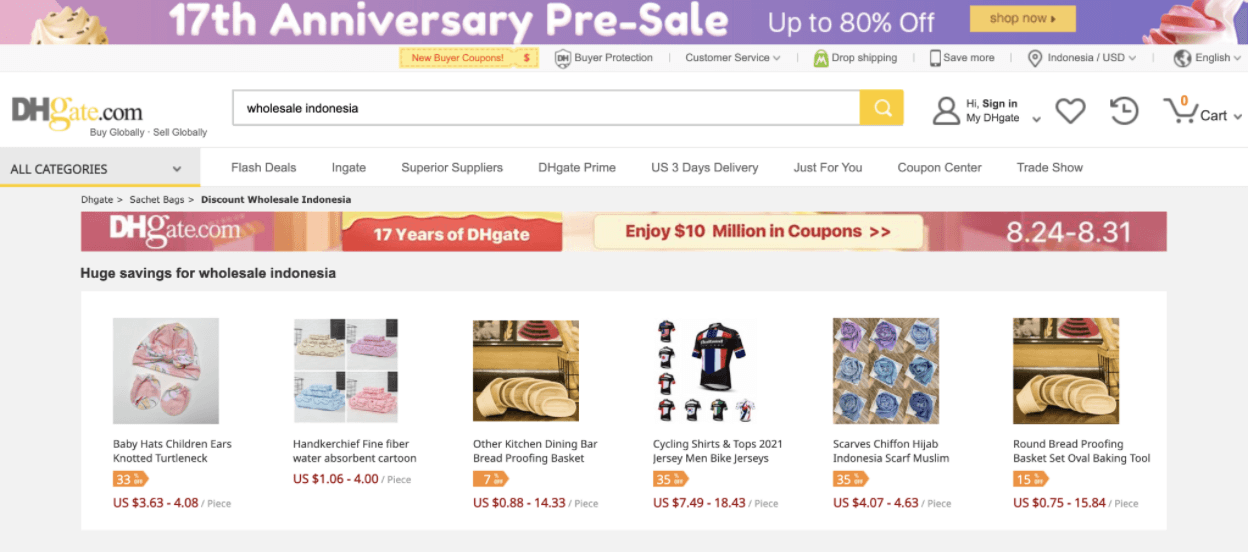### Descriptive Caption:
The image is a vibrant advertisement for DH Gate's 17th anniversary pre-sale. At the top, a purple banner prominently displays "17th Anniversary Pre-Sale" in bold white text, alongside "Up to 80% Off," also in white. A striking yellow "Shop Now" button provides a call to action. The corners of the banner are whimsically decorated with ice cream graphics, adding a playful touch.

Beneath the top banner, a yellow square with red text offers a new buyer coupon, emphasizing savings. Additional features like buyer protection, customer service, and drop shipping options are highlighted, catering specifically to customers in Indonesia and English-speaking markets.

Further down, the DH Gate logo appears, with 'DH' in black and 'Gate' in yellow, followed by '.com'. The tagline "Wholesale Indonesia" underscores the platform's focus. A small person icon indicates the sign-in option, enhancing user accessibility.

Showcased below are six different products under the headline "17 Years of DH Gate," emphasizing bulk purchasing opportunities. The promotion boasts an enticing offer, inviting users to "Enjoy $10 Million in Coupons."

This detailed layout and vibrant design effectively communicate the extensive savings and benefits available during the anniversary sale.